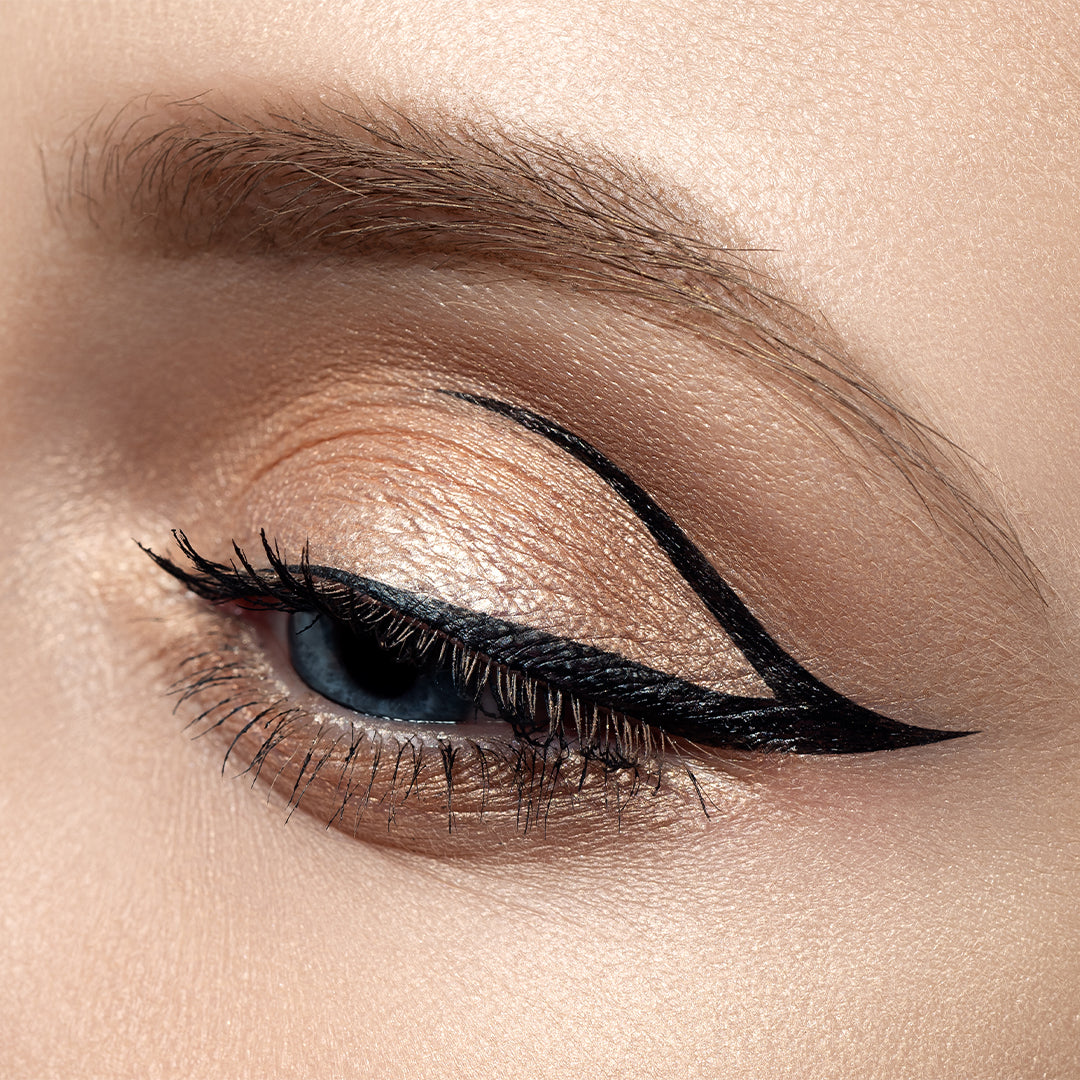This image features a close-up of a woman's left eye and the surrounding area. The focal point is her well-made-up eye, which is light blue. She wears a striking combination of black eyeliner and mascara. The eyeliner is applied both along the upper lash line and in a distinctive 'V' shape that extends outward and upward at the corner of her eye, giving a dramatic cat-eye effect. Additionally, her eyelids are adorned with a blend of gold and bronze eyeshadow, accentuating her eye color. Her eyebrows are neatly groomed and filled in, complementing the intricate makeup. The upper part of her cheek and a portion of her forehead, along with her brown hair, frame the eye, set against her delicate, pinkish flesh tone. This detailed makeup possibly draws inspiration from high fashion, highlighting innovative cosmetic techniques.